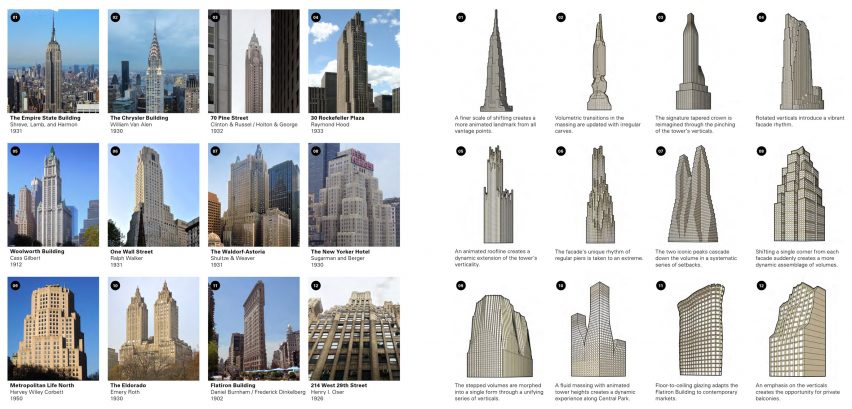The image consists of two adjacent squares. The left square features twelve photographs of iconic New York City skyscrapers, arranged in three rows and four columns. These photographs capture the upper portions of the buildings against clear blue skies, with about the bottom 20% cropped out. The buildings include (from top left to bottom right): the Empire State Building, the Chrysler Building, 70 Pine Street, 30 Rockefeller Plaza, the Woolworth Building, 1 Wall Street, the Waldorf Astoria, the New Yorker Hotel, Metropolitan Life North, the Eldorado, the Flatiron Building, and 214 West 28th Street.

Each photograph has a small black circle in the upper left corner containing a number. On the right side of the image, the square mirrors the arrangement of the left square but features outlined sketches of the same buildings instead of photographs. The backgrounds of these sketches are plain white, and the buildings are rendered in simple lines. Below each sketch, there are two or three lines of text, though the text is too small to read. These sketches also have black circles with numbers in the upper left corners, corresponding to the photographs on the left.